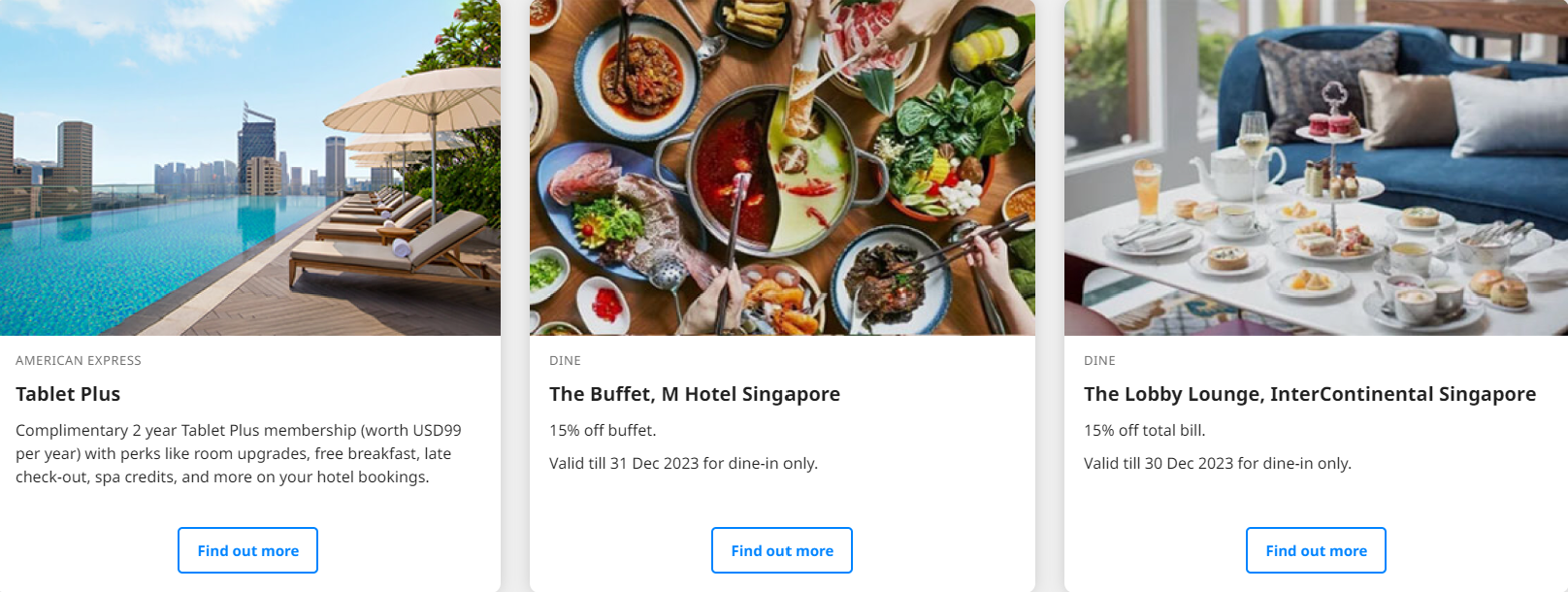### Image Descriptions:

1. **Luxury Poolside Retreat**: The first image captures a serene poolside setting, perfect for relaxation. In the foreground, there are inviting deck chairs and beach umbrellas, indicating a prime spot to unwind. The backdrop features a stunning city skyline, adding a touch of urban sophistication to the scene. Below the image, "American Express" is prominently displayed, promoting a special offer: a complimentary two-year Tablet Plus membership worth US $99 per year. This membership includes perks such as room upgrades, free breakfasts, late checkouts, spa credits, and more on hotel bookings. There's also a "Find out more" button for additional details.

2. **Gourmet Dining Experience**: The second image is an overhead shot of a communal dining setup, brimming with various dishes. Multiple hands are visible, reaching in with utensils and chopsticks to sample the diverse offerings. This lively scene signifies a buffet dining experience. The caption mentions "The Buffet, M Hotel Singapore," and highlights a special offer of 15% off the total bill, valid until 31 December 2023 for dine-in only. A "Find out more" button provides further information.

3. **Elegant Dining Room Setting**: The final image shows a sophisticated dining room adjacent to a window, suggesting a bright, airy atmosphere. The room features a plush sofa with three decorative throw pillows, and a pristine white table set with multiple gourmet dishes, a tiered tray, and an assortment of drinks including champagne and beers, evoking a high-class dining experience. The caption indicates "The Lobby Lounge, Intercontinental Singapore," and advertises a 15% discount on the total bill, valid until 30 December 2023 for dine-in only. A "Find out more" button is available for those interested.